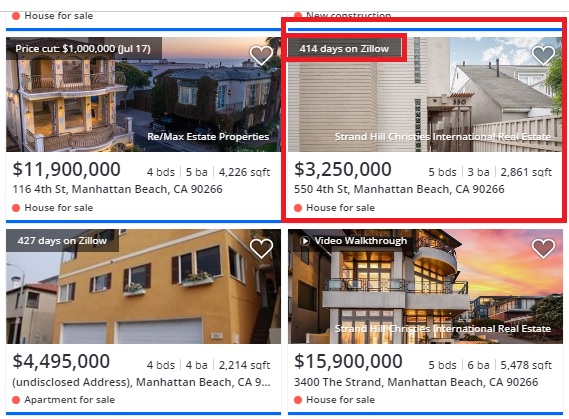Screenshot Description: Housing Listings Near Manhattan Beach, California

This screenshot captures a selection of property listings from a housing website, all situated in the desirable area of Manhattan Beach, California. The listings primarily feature houses for sale, many of which are marked as new constructions.

**Details of Listings:**

1. **Top Left**:
   - **Real Estate Agency**: REMAX Estate Property
   - **Price**: $11,900,000 (recent price cut of $1 million on July 17th)
   - **Features**: 4 bedrooms, 5 bathrooms, 4,226 square feet
   - **Location**: Manhattan Beach, California

2. **Bottom Left**:
   - **Property Type**: Apartment
   - **Time on Zillow**: 727 days
   - **Price**: $4,495,000
   - **Features**: 4 bedrooms, 4 bathrooms, 2,214 square feet

3. **Top Right (Circled in Red)**:
   - **Chosen Property**
   - **Price**: $3,250,000
   - **Time on Zillow**: 414 days
   - **Features**: 5 bedrooms, 3 bathrooms, 2,861 square feet

The detailed listing information, including prices, features, and time on Zillow, paints a comprehensive picture of the housing options available in Manhattan Beach. The circled property at the top right signifies the user's selection, highlighting its competitive pricing and spacious layout.